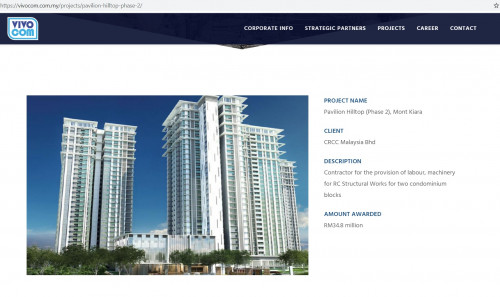This is an image of a website interface that appears to be somewhat difficult to read due to small lettering. The top portion of the page features a thin, light gray area, which likely displays the website's address, although it is not legible. Below this is a section that is either black or navy blue in color. On the left side of this darker section, there is a bubble-like graphic that is white and outlined in blue, containing the words "Vivo.com" in two shades of blue.

Centrally positioned on the darker section, extending towards the right, there are clickable options labeled as follows: "Corporate Info," "Strategic Partners," "Projects," "Career," and "Contacts."

Moving further down, the background transitions to a large white area. Within this section, there is a square image featuring at least three, potentially four, tall buildings standing against a blue sky dotted with green trees. To the right of this image, there are text elements, although difficult to read, that likely consist of a project name, client information, a description of the project, and the amount awarded for the project.